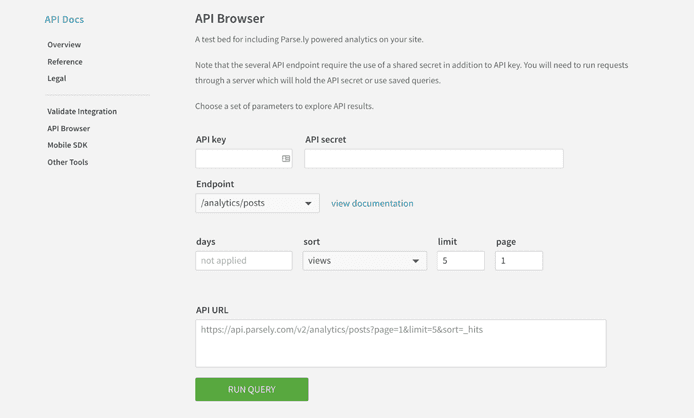Screenshot Description:

The screenshot features a predominantly light gray background showcasing an API interface. On the left sidebar, highlighted in blue, the section title reads "API Docs" with subcategories listed below: "Overview," "Reference," "Legal," followed by a gray separator line. Additional options such as "Validate Integration," "API Browser," "Mobile SDK," and "Other Tools" appear further down.

In the main content area, the page is titled "API Browser" in bold text at the top. Below the title, the description reads: "A testbed for including Parse.ly-powered analytics on your site. Note that several API endpoints require the use of a shared secret in addition to an API key. You will need to run requests through a server which will hold the API secret or use saved queries. Choose a set of parameters to explore API results."

There are input fields for "API Key" and "API Secret," both currently empty. An endpoint selection dropdown menu displays "slash analytics slash posts," accompanied by a blue, likely hyperlinked text labeled "View Documentation" to its right. 

Further down, a series of parameter input fields include:
- "Days," with an input box containing light gray placeholder text that reads "not applied"
- "Sort," with a dropdown box set to "views"
- "Limit," with a box set to "5"
- "Page," with an input box set to "1"

An API URL is detailed below these parameters: "https://api.parsely.com/v2/analytics/post?page=1&limit=5&sort=_hits."

At the very bottom, a prominent green button with white, all-caps text reads "RUN QUERY."